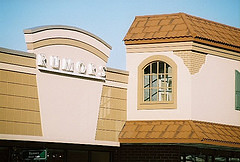The image captures the top section of a storefront called "Roomers," situated in a public place, potentially a restaurant or shop, under a vibrant daytime sky. The structure is predominantly beige, with the name "Roomers" displayed prominently in white capital letters on a cream-colored, slightly triangular facade with a flat bottom and rounded top. Adjacent to this central section is another part of the building featuring a crow's nest-like structure with a large half-circular window and brown slats, further complemented by a brown tiled roof that descends to a beige base. The expansive, clear blue sky serves as the backdrop, accentuating the storefront's colors and design details. At the image's bottom edge, the top of the building's doors is faintly visible along with an indistinct sign, adding to the public and welcoming ambiance of the place.